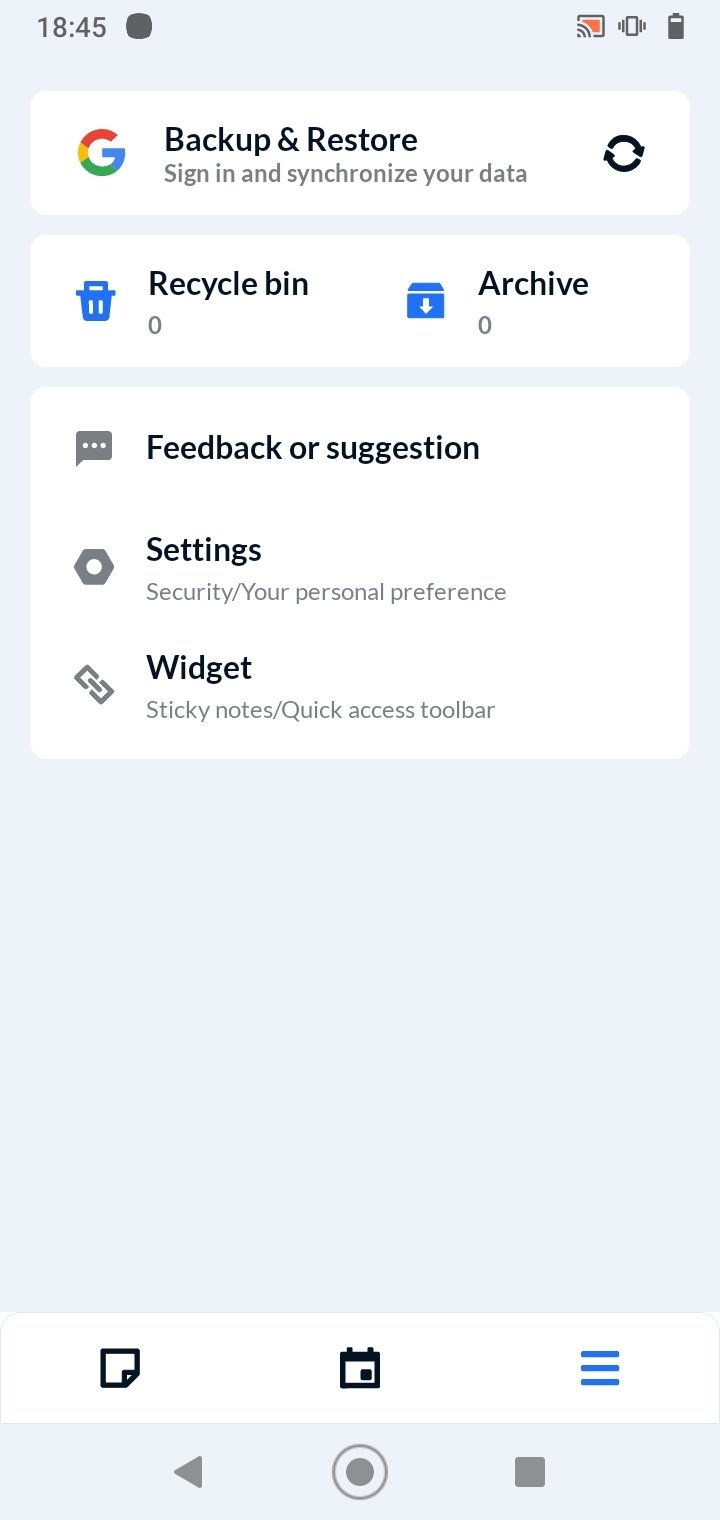The image depicts a user interface screen divided into several sections. 

- At the top left corner, a light gray box features the number "1845" prominently. 
- Opposite on the top right, a battery icon is displayed, indicating the device's battery status. 

Beneath this top panel, there is a white box with the Google logo prominently positioned. Next to the logo, the text reads: "Backup and Restore - Sign in and synchronize your data". The text is accompanied by an icon of two arrows forming a circle, symbolizing synchronization.

Following this, another section contains a blue trashcan icon labeled "Recycle Bin - 0", indicating that the recycle bin is empty. Adjacent to this, there is a blue box labeled "Archive - 0", similarly indicating that the archive is empty.

Further down, a larger white box includes a gray text box with an ellipsis inside. This section is labeled "Feedback or Suggestions", presumably inviting users to provide input.

Below this, a hexagonal shape with a hole in the center is labeled "Settings - Security / Your Personal Preference", likely a button to access a settings menu.

The final section displays a gray background and contains the text "Widget - Sticky Notes / Quick Access Toolbar", indicating the presence of customizable tools for user convenience.